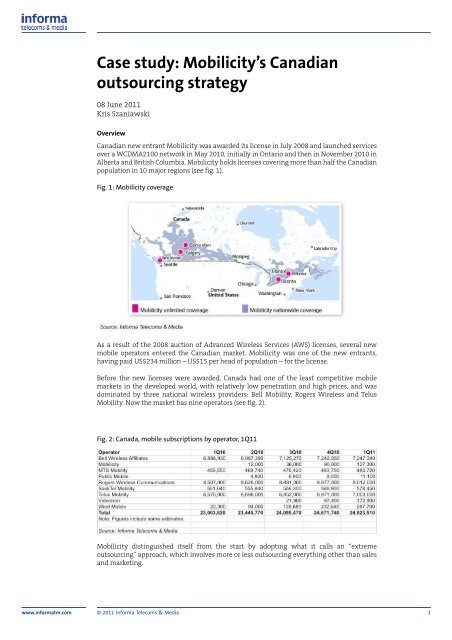This image is of a page taken from a case study by Informa Telecoms and Media, titled "Mobilicity's Canadian Outsourcing Strategy", authored by Chris Sazweski (June 8, 2011). At the top left corner, the name "Informa Telecoms and Media" is visible in blue. The page includes several sections such as an overview, a map illustration, and a table. The map highlights Mobilicity's coverage in Canada with pink dots indicating specific areas and purple shading representing nationwide coverage. Despite the blurred print making most of the text hard to read, it's noted that this is page one of the case study which was published in 2011. There is a color code at the bottom of the map and additional data, including "Canada Mobile Subscription by Operators" for the year 2011, is mentioned. The website is also visible at the bottom left corner of the page.